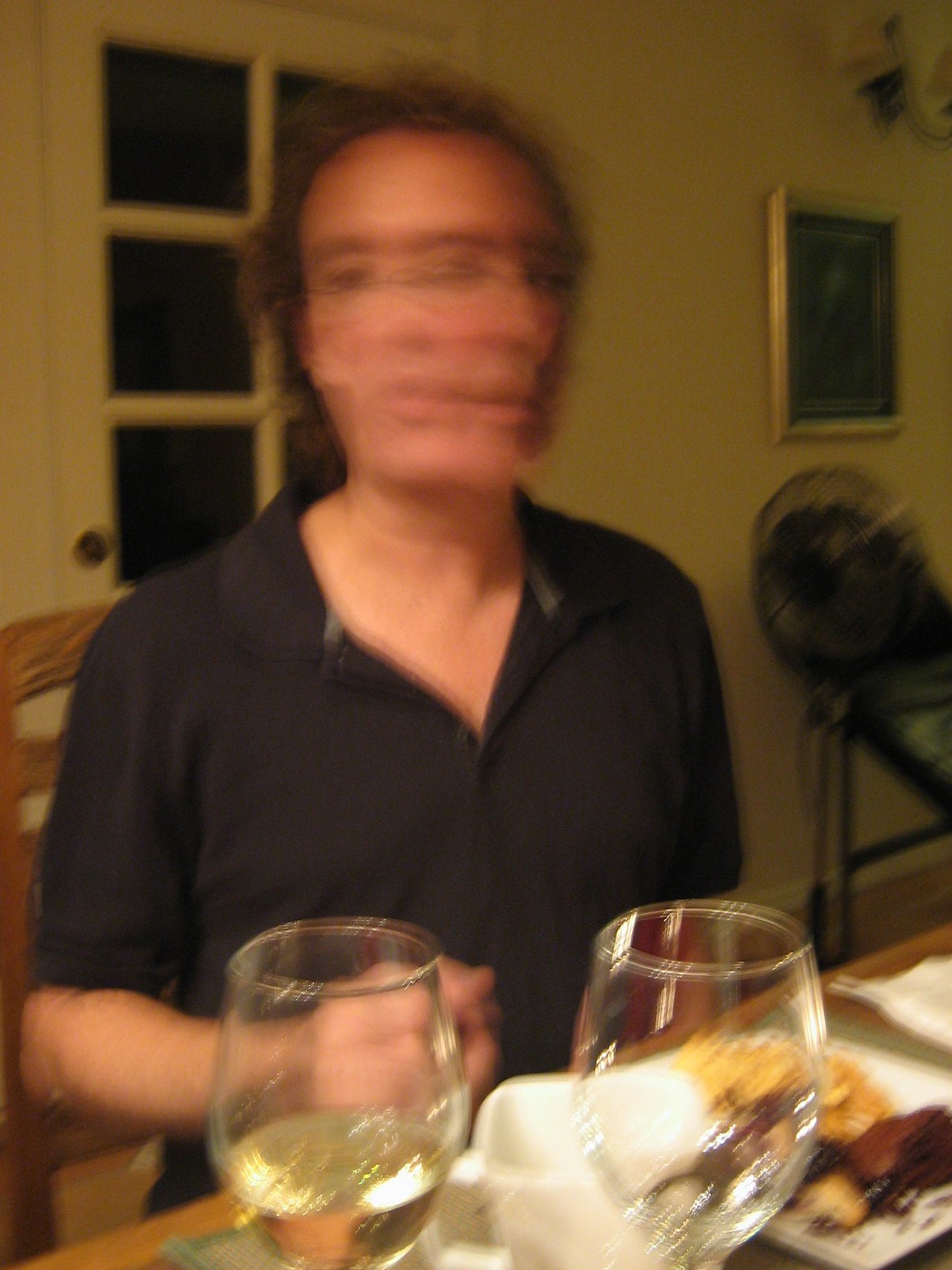In this blurry image, a man is seated at a table, his head in motion as though he is turning it side to side, making his head the blurriest part of the photo. The man has short, somewhat curly brown hair and wears a black short-sleeve shirt with a collar and a few buttons at the front, the top two or three of which are undone. His right arm is bent, with his hand resting on the table. There are two wine glasses in the foreground, closest to the camera. The wine glass on the left contains a small amount of wine, while the one on the right appears to be empty.